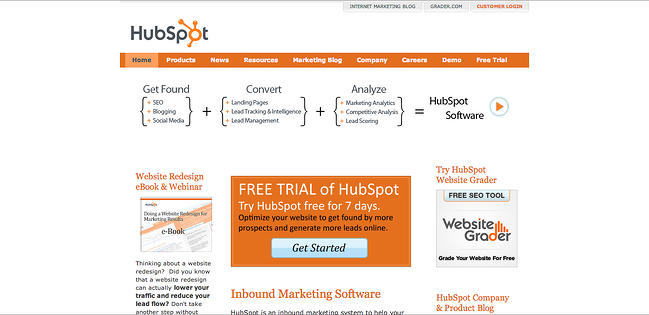This is an image from HubSpot’s website featuring a detailed layout and branding elements. At the top, an orange section spans the width of the image, prominently displaying the word "home," which is illuminated, indicating the current page. Beneath this, in bold black text, it lists the core functionalities of HubSpot with the phrase: “Get Found + Convert + Analyze = HubSpot Software.”

The HubSpot logo is creatively designed with “H-U-B-S” in black letters, while the "O" is represented as an orange circular icon with radiating lines ending in orange balls. The "T" remains in black, seamlessly integrating with the rest of the logo.

To the right, there is a circular icon with an orange arrow indicating an interactive element where users can click to watch a video for more information. Below this icon, the text reads "Website Redesign E-book and Webinar," accompanied by an image of an e-book.

Centrally positioned, the text promotes a free trial of HubSpot with a compelling call-to-action: "Free Trial of HubSpot. Try HubSpot free for seven days." Below this, a blue button with black letters invites users to “Get Started.”

Adjacent to the central text, another section highlights HubSpot’s free SEO tool, displayed as "Free SEO Tool. Try HubSpot Website Grader." It features a boxed text where “Website Grader” is displayed, with the "D" in "Grader" colored orange, followed by two orange lines.

Towards the bottom, partially visible text mentions "Inbound Marketing Software" and continues with "HubSpot Company and Product Blog," though this section is somewhat cut off.

Overall, the image offers a comprehensive overview of HubSpot’s diverse marketing tools and resources, effectively engaging the user with clear calls to action and an inviting layout.